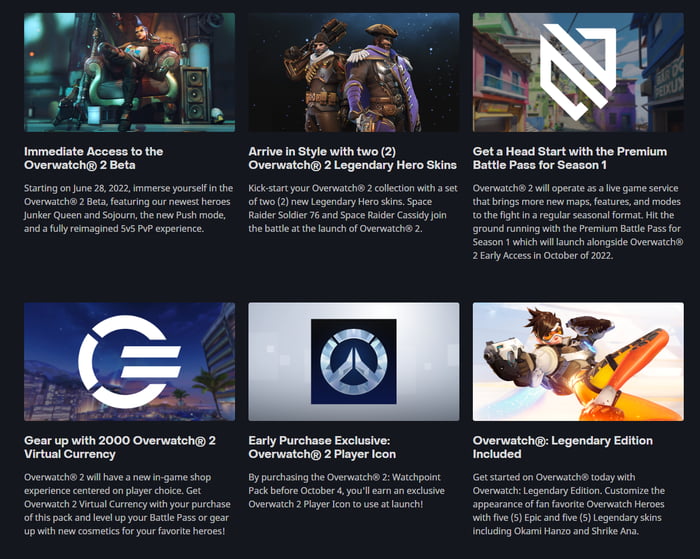This webpage, featuring a sleek black background, is divided into two rows of three images, forming a grid that highlights various aspects of the video game Overwatch 2.

1. **Top Row, Image 1:** The first image showcases Junker Queen, a punk rock Australian woman, seated confidently on a throne. The caption reads: "Immediate access to the Overwatch 2 beta starting on June 28, 2022. Immerse yourself in the Overwatch 2 beta featuring our newest heroes Junker Queen and Sojourn, the new push mode, and a fully reimagined 5v5 PvP experience.”

2. **Top Row, Image 2:** This image displays two iconic Overwatch characters, Reaper and Cassidy. The text reads: "Arrive in style with two Overwatch 2 legendary hero skins. Kickstart your Overwatch 2 collection with a set of two new legendary hero skins: Space Raider Soldier 76 and Space Raider Cassidy. Join the battle at the launch of Overwatch 2.”

3. **Top Row, Image 3:** The final image in the top row depicts a map resembling a Brazilian favela, accompanied by the caption: "Get a head start with the premium battle pass for season one. Overwatch 2 will operate as a live game service offering new maps, features, and modes in a regular seasonal format. Launching alongside Overwatch 2 early access in October 2022.”

**4. Bottom Row, Image 1:** An image of a cityscape under a dark sky with a unique icon in the middle. The caption states: "Gear up with 2000 Overwatch 2 virtual currency. Overwatch 2 will feature a new in-game shop centered on player choice. Use the Overwatch 2 virtual currency to level up your battle pass or acquire new cosmetics for your favorite heroes.”

**5. Bottom Row, Image 2:** Featuring the Overwatch logo in silver against a black background, the text reads: "Use the early purchase exclusive Overwatch 2 player icon. By purchasing the Overwatch 2 Watchpoint Pack before October 4, you earn an exclusive Overwatch 2 player icon to use at launch.”

**6. Bottom Row, Image 3:** The final image portrays Tracer in her default uniform aiming at the camera. The accompanying text reads: "Overwatch Legendary Edition included. Get started on Overwatch today with the Overwatch Legendary Edition, which includes five epic and five legendary skins, including Okami Hanzo and Shrike Ana.”

This detailed layout effectively markets the new features and upcoming content in Overwatch 2, enticing fans with exclusive beta access, new hero skins, in-game currency, and various other enhancements.